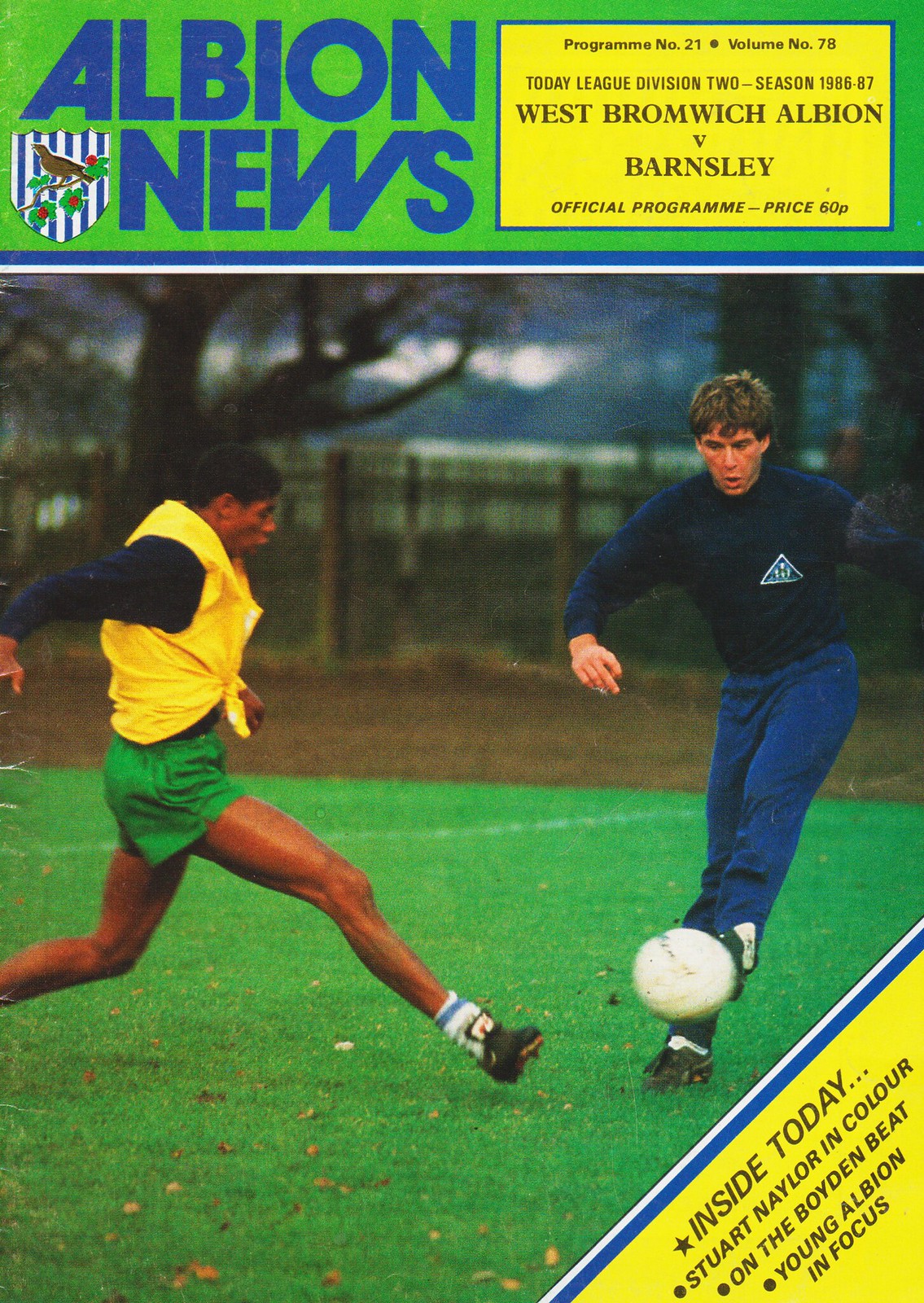The image depicts the front cover of a historical football programme titled "Albion News" from the 1986-87 season. The top portion of the cover features a green banner, with "Albion News" prominently displayed in blue block capitals on the left and a white and blue crest with a bird roosting on a branch in the center. To the right, within a yellow rectangle outlined in blue, the text reads: "Program Number 21, Volume Number 78, Today League Division Two, Season 1986-87, West Bromwich Albion vs. Barnsley, Official Programme, Price 60p." Below, a color photograph captures the dynamic scene of a soccer match. On the left, a black male player with short afro hair is pictured wearing green shorts, a yellow vest, and a long-sleeve blue shirt, poised to kick the ball. On the right, a white male player with short brown hair is seen in blue pants and a blue long-sleeve shirt, controlling the ball. The green soccer field extends into the distance, bordered by wooden fencing and interspersed with trees. In the bottom right corner, a yellow triangle announces: "Inside Today: Stuart Naylor in color, On the Boyden Beat, Young Albion in Focus."